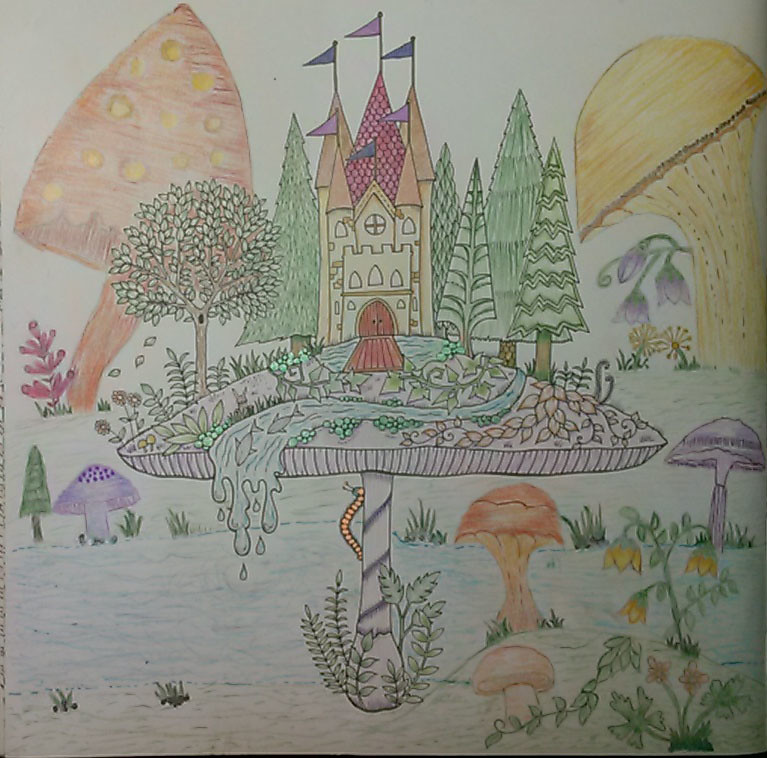This color photograph showcases an intricately detailed, hand-drawn artwork, likely created using colored pencils. The drawing centers around a grand castle perched atop a large, round mushroom cap that spans the middle of the frame. The castle features five spires adorned with six flags in shades of purple and blue, a red main door, and a few scattered windows. Surrounding the castle are tall pine trees and a couple of leafed trees, painted in pastel shades of green.

A small stream originates from the castle and flows across the mushroom cap, culminating in a waterfall that cascades over the edge, where two fish are seen about to tumble off. An orange worm or caterpillar is depicted crawling up the mushroom stem, adding a whimsical touch to the scene. 

The foreground of the composition features a blue sea and grass dotted with multicolored mushrooms in hues of purple, red, yellow, and orange. These mushrooms, varying in size and placement, enhance the fantastical and childlike yet sophisticated charm of the artwork. A yellow mushroom and an orange tree with yellow fruit, both tilting towards the castle, further enrich the background, accentuating the fairy-tale ambiance of the piece.